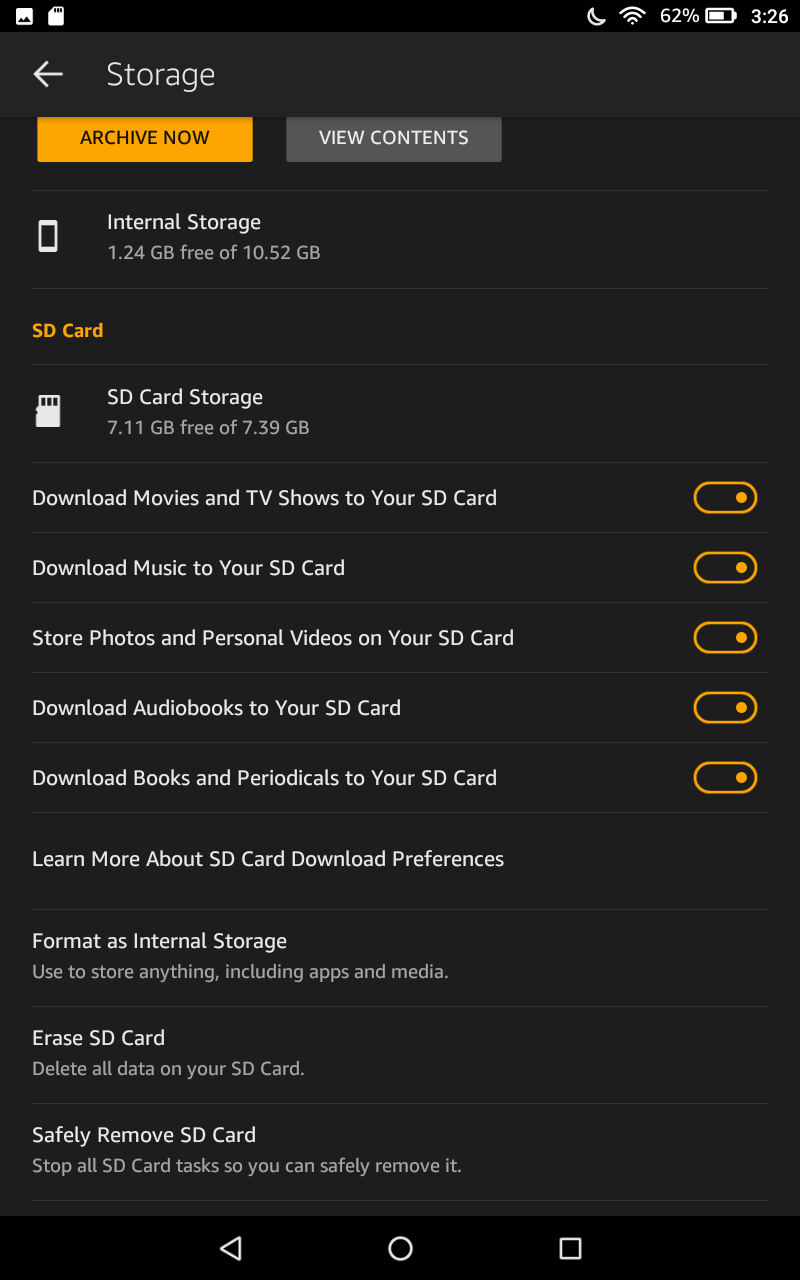This image is a detailed screenshot of a mobile device's storage settings interface. At the top of the screen, the status bar displays multiple icons against a black background. On the far left, there are white square icons, followed by a crescent moon icon, the Wi-Fi symbol, and the battery icon showing 62% remaining power. The time is indicated as 3:26. Below the status bar, a back arrow symbol occupies the upper-left corner.

The primary interface features two central sections highlighted in distinct colors. The first section is an orange and black box labeled "Archive Now," and the adjacent section is a white and gray box labeled "View Contents." 

Further down, a graphic resembling a white cell phone icon is shown next to the internal storage status: **"Internal Storage: 1.24 GB free of 10.52 GB."** Below that, an orange section with a white SD card graphic displays the external storage status: **"SD Card Storage: 7.11 GB free of 7.39 GB."**

Subsequently, there are listed actions associated with an orange box, indicating options available for the SD card:
- **Download movies and TV shows to your SD card**
- **Download music to your SD card**
- **Store photos and personal videos in your SD card**
- **Download audiobooks to your SD card**
- **Download books and periodicals to your SD card**

Following these options, additional sections do not have orange boxes and include:
- **Learn more about SD card download preferences**
- **Format as internal storage**
- **Store anything including apps and media**
- **Erase SD card (delete all data on your SD card)**
- **Safely remove SD card (stop all SD card tasks so you can safely remove it)**

At the bottom of the screen are three navigation icons: a back triangle, a white circle, and a white square, indicating navigation controls for the device.